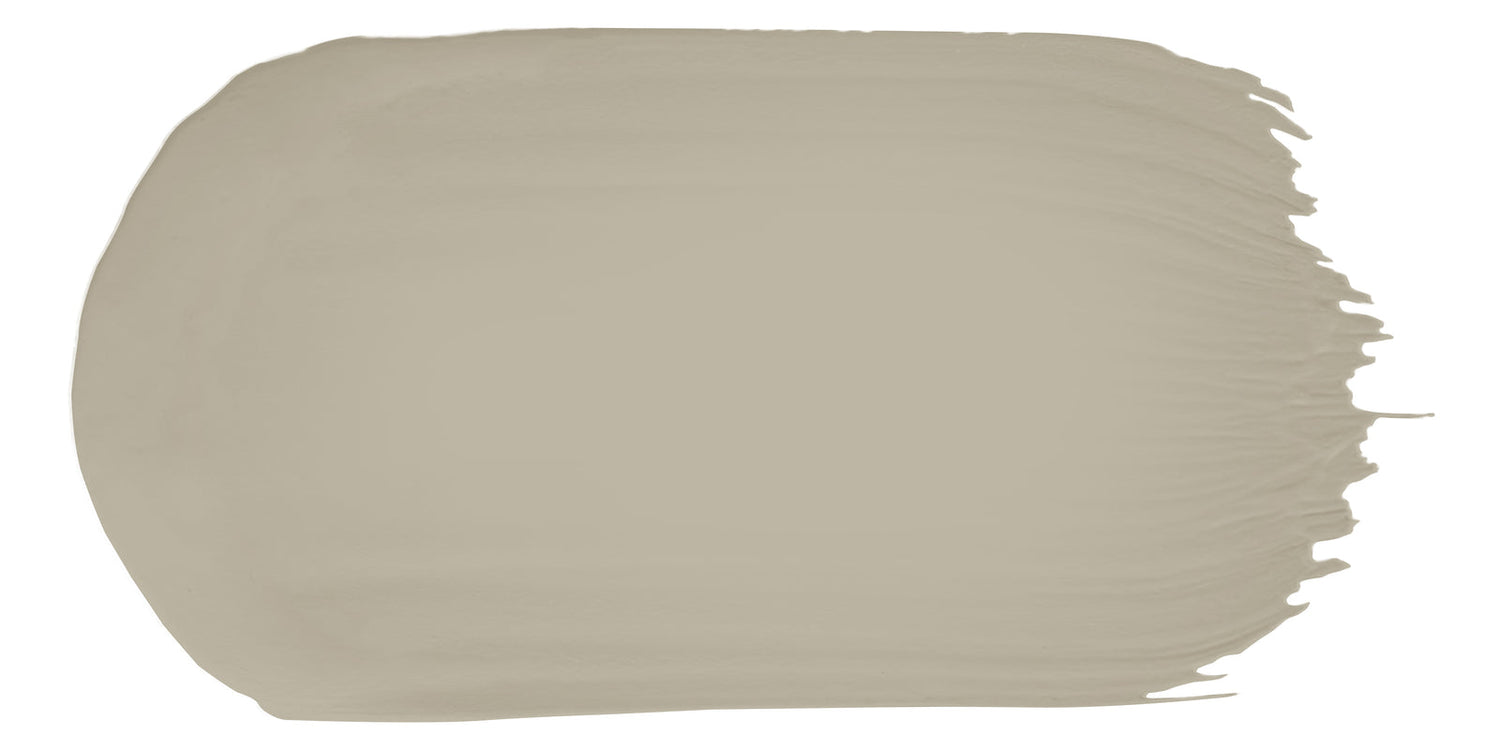The image depicts a modernistic stroke of paint against a white background. The paint is a medium or slate gray color, possibly resembling taupe. The shape is somewhat oblong, with a smooth, rounded left side that curves like a capsule. The top and bottom edges are straight, while the right edge is jagged and uneven, as if the paintbrush was lifted abruptly, leaving a smeared, textured trail. The figure possesses a subtle texture, indicative of oil paint, providing a slightly tactile appearance amidst its otherwise smooth and orderly form.